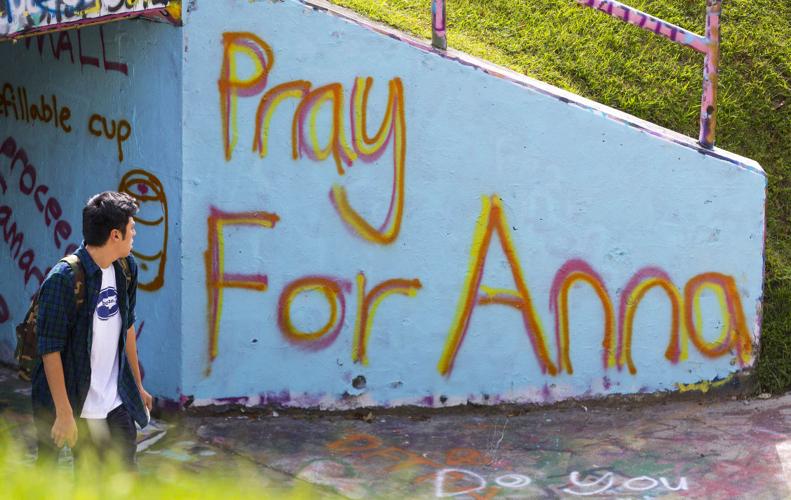A young Caucasian man with dark hair, possibly in his mid-20s, is captured in this photo walking near an underpass during the daytime. The concrete walls of the underpass are covered with various graffiti. Prominently featured on the sloping side wall is a large spray-painted message that reads in red and yellow letters, "Pray for Anna." The man, who is wearing a backpack, a white t-shirt, and a blue flannel shirt with the sleeves rolled up, appears to be looking at this message. He is seen emerging from the underpass, with his face turned to his left, which is to the right in the picture. Behind him, there are additional writings, including phrases such as "Do You" on the ground and other words in reddish letters further inside the underpass. The top of the wall features metal posts and beyond it, there is greenery on a hillside. The underpass seems to lead toward a bridge over a road, suggesting a somewhat urban setting. The detailed graffiti, along with the presence of the man who may have just finished painting, enriches the narrative of the scene.